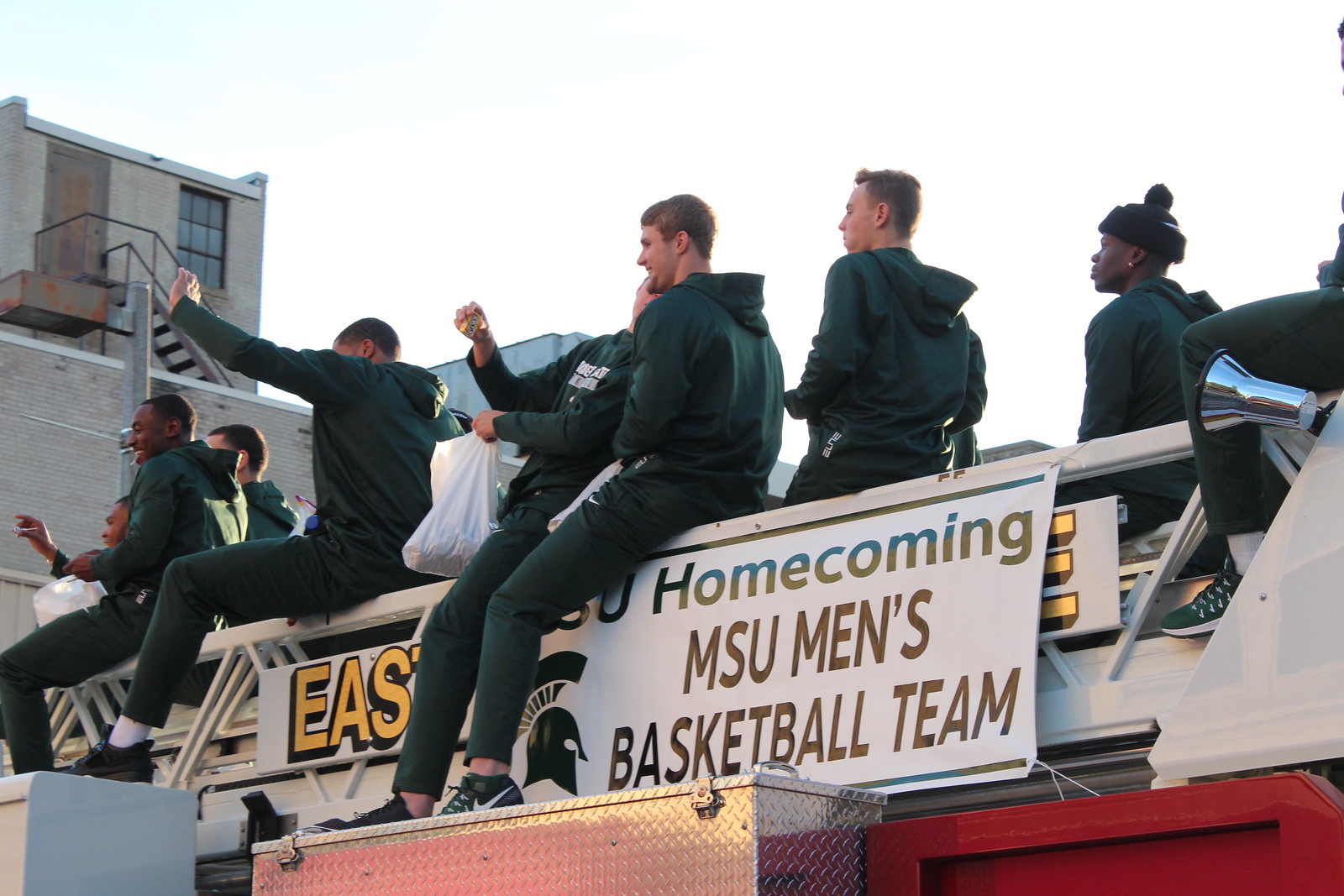The image depicts nine men riding on top of a fire truck, likely part of a parade or celebratory procession. These men, possibly members of the MSU Men's Basketball Team, are sitting on the ladder of the fire truck, dressed in athletic gear such as hoodies and sweatpants. They are waving and appear to be engaging with the crowd, with one man likely distributing candy from a bag. The vehicle features a sign that reads "Homecoming MSU Men's Basketball Team," accompanied by a logo of a gladiator helmet with a plume. Visible in the background is a building with stairs, windows, and a door, along with a blocked-off sign that partially reads "East." The setting is outdoors on a clear day, presumably on a parade route, amid a backdrop of white, light blue, brown, light brown, green, yellow, silver, and red colors. The fire truck’s distinctive red body and chrome supply boxes are also prominently visible.